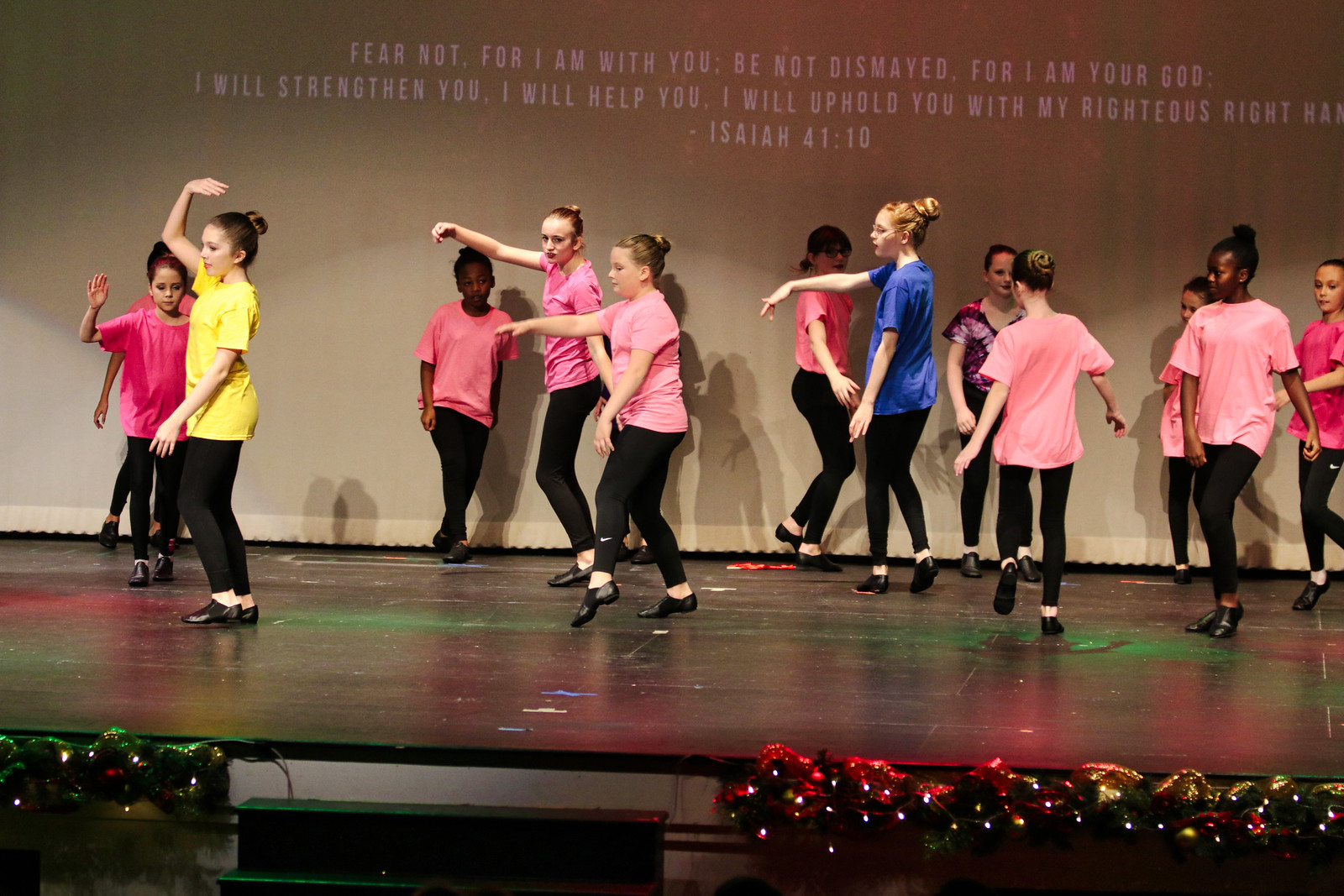The image captures a vibrant dance performance on a predominantly black stage featuring a group of young girls. These girls are attired in black tights and black ballet or tap shoes, each donning a colorful short-sleeve t-shirt; pink, blue, and yellow are clearly visible. Their hair is uniformly styled in buns, adding a touch of elegance to their coordinated movements. The backdrop includes a large, tan curtain with a projected religious quote from Isaiah 41:10, which reads, "Fear not, for I am with you. Be not dismayed, for I am your God. I will strengthen you, I will help you, I will uphold you with my righteous right hand." The stage itself is wooden and adorned with colorful bows and twinkling Christmas lights on either side, adding a festive touch. In the foreground, steps lead up to the stage, further enriching the scene. The girls dance gracefully, some on tiptoes and others using expressive hand gestures, creating a lively and engaging atmosphere.